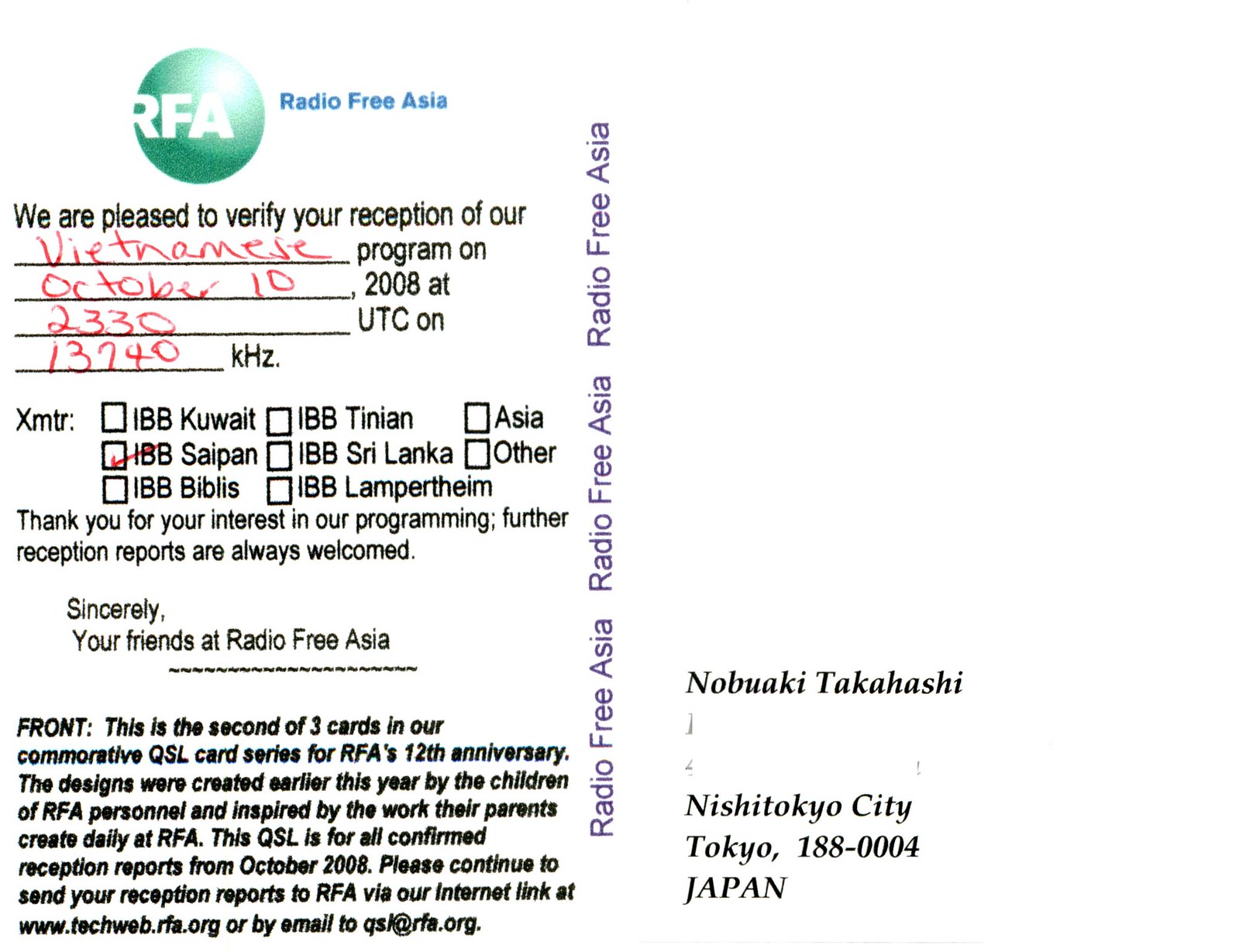This image depicts a commemorative QSL postcard from Radio Free Asia against a white background. Dominating the top section is a green circle with the Radio Free Asia logo, accompanied by the text "Radio Free Asia" in blue print. The main body of the card features a formal verification message stating, "We are pleased to verify your reception of our Vietnamese program on October 10th, 2008, at 2330 UTC on 13740 kHz." This text is handwritten in red ink to fill in the specified details. The card further extends gratitude for the recipient's interest in the programming, signed sincerely by "your friends at Radio Free Asia," encouraging future reception reports.

On the right side, the recipient's address is included, identifying the individual as Nabuaki Takahashi from Nishitokyo City, Tokyo, Japan, with a partial whiting out of the address, leaving "Tokyo 188-0004, Japan" visible. Additional information on the card includes that it is the second of three in a commemorative series celebrating RFA's 12th anniversary, with designs created by children of RFA personnel.

The color scheme includes white, green, blue, black, red, and purple, with the postcard itself filling the entire image frame, suggesting it was photographed or scanned for record-keeping or presentation purposes.